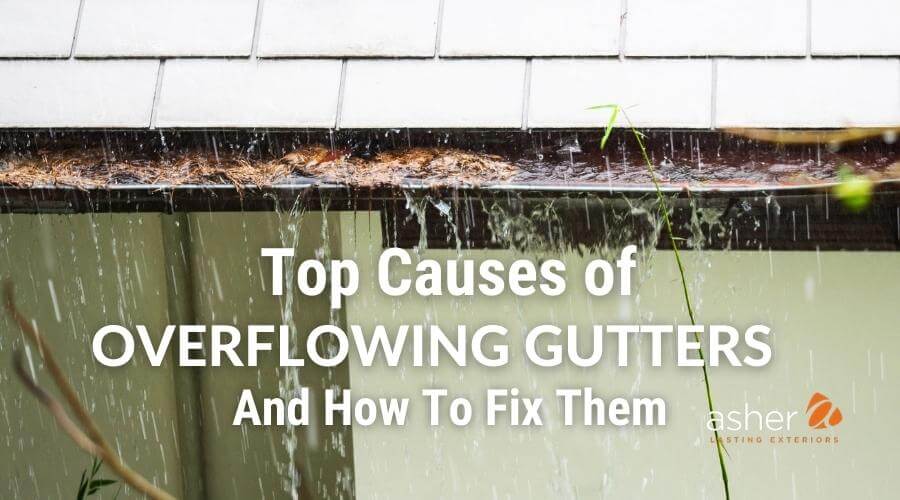The image is an advertisement-style outdoor shot of a house's gutter and roof area amidst a rainstorm. At the top, white shingles are visible, with rain cascading down into a gutter filled with brown pine needles. The gutter, featured prominently, runs horizontally across the image. Below the gutter, the house's siding is observable, with an olive tone on the left and a lighter olive or grayish tint on the right. Framing the scene are vertical running boards. Overlaying the image in white text near the center bottom are the words: "Top causes of overflowing gutters and how to fix them." In the bottom right corner, there's a logo consisting of an orange A within a triangle, accompanied by the text "Asher" in white and "lasting exteriors" in smaller orange font below.